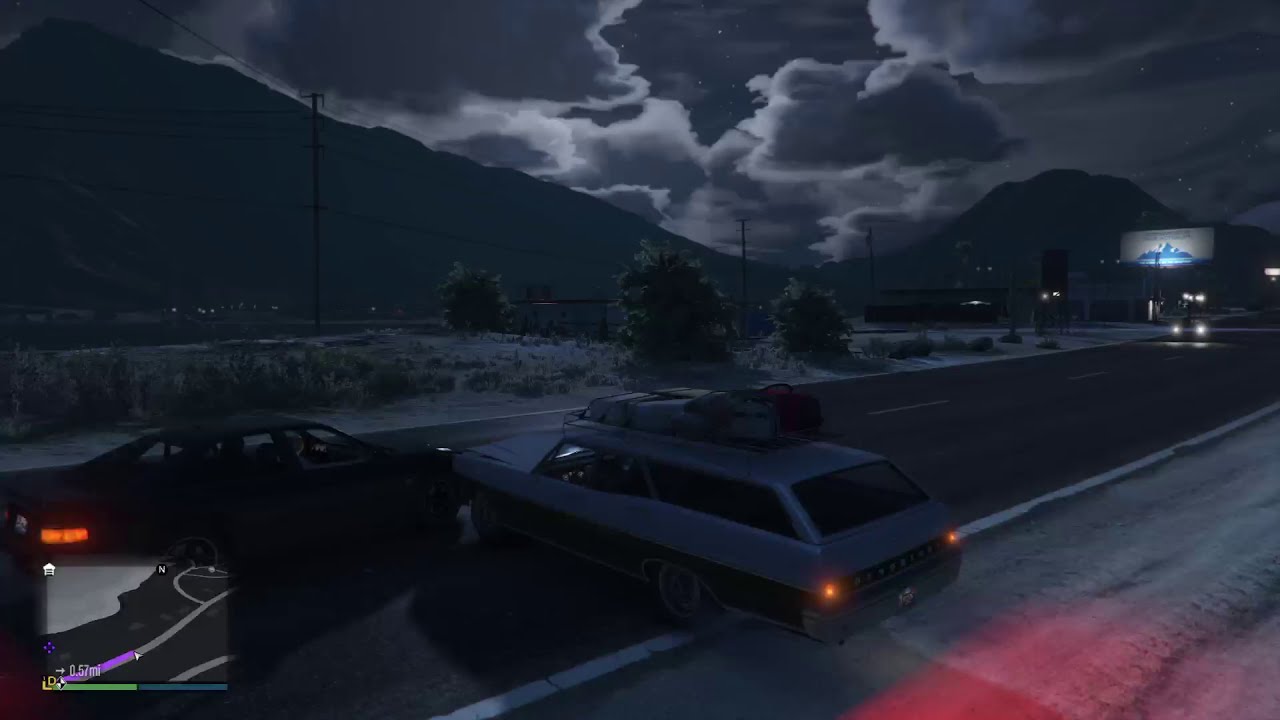The scene is set at nighttime in a desolate, outdoor environment, likely from the video game GTA. The sky is filled with grayish puffy clouds, and a mountain range looms in the background, with a peak on the left and another on the far right. Below these mountains, a lit white sign features a blue mountain graphic, and to the right are some colored lights, possibly from buildings or light poles.

In the foreground, two cars have collided perpendicularly on a single lane, black road. The road, with dashed white center lines and solid white side lines, runs from the lower left to the middle right of the image. One car, resembling a minivan or hybrid vehicle, is partially off the road on its back two wheels. The other car, a black coupe with red brake lights, sits to the left of it. A third car, with its headlights on, approaches from the middle right.

To the bottom left of the image, a detailed map shows the player's location and direction within the game, marked by a purple line indicating the route. The map also features a driving point and a white house icon on the top left, with yellow and blue bars beneath. The surroundings include tan sand, sparse green bushes, and several brown telephone poles. A blue and white billboard and a building are visible on the right side of the image, adding to the desolate nighttime setting.